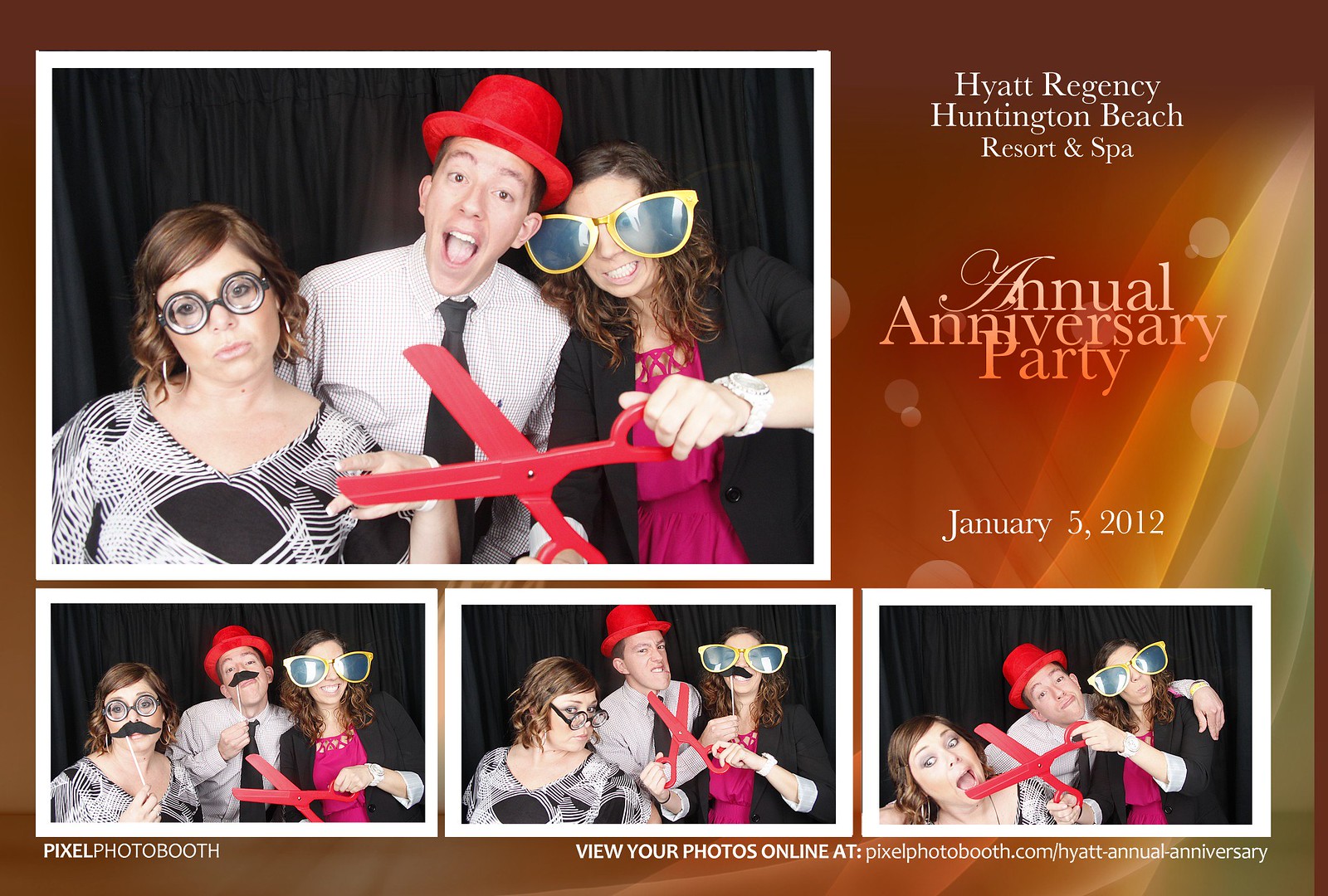This descriptive caption consolidates the details from all three inputs:

The flyer for the Hyatt Regency Huntington Beach Resort and Spa announces their Annual Anniversary Party on January 5, 2012, with an attractive gold background featuring radiating gold rays. At the top right, white lettering reads "Hyatt Regency Huntington Beach Resort and Spa". On the left, it says "Annual Anniversary Party" with the date underneath. The large central photo, framed in white, showcases three young people: on the left is a girl in a black dress with white lines and funny glasses, in the center is a boy wearing a white shirt, black tie, and a red hat, and on the right is another girl with oversized glasses and toy pink-red scissors, dressed in a maroon dress and short jacket. Below the primary image are three smaller photos of the same trio in varying poses. At the bottom, against a dark brown-gold background, the text reads "Pixel Photo Booth. View your photos online at pixelphotobooth.com/Hyatt-Annual-Anniversary". These lively images and playful costumes likely depict employees having fun at the event.